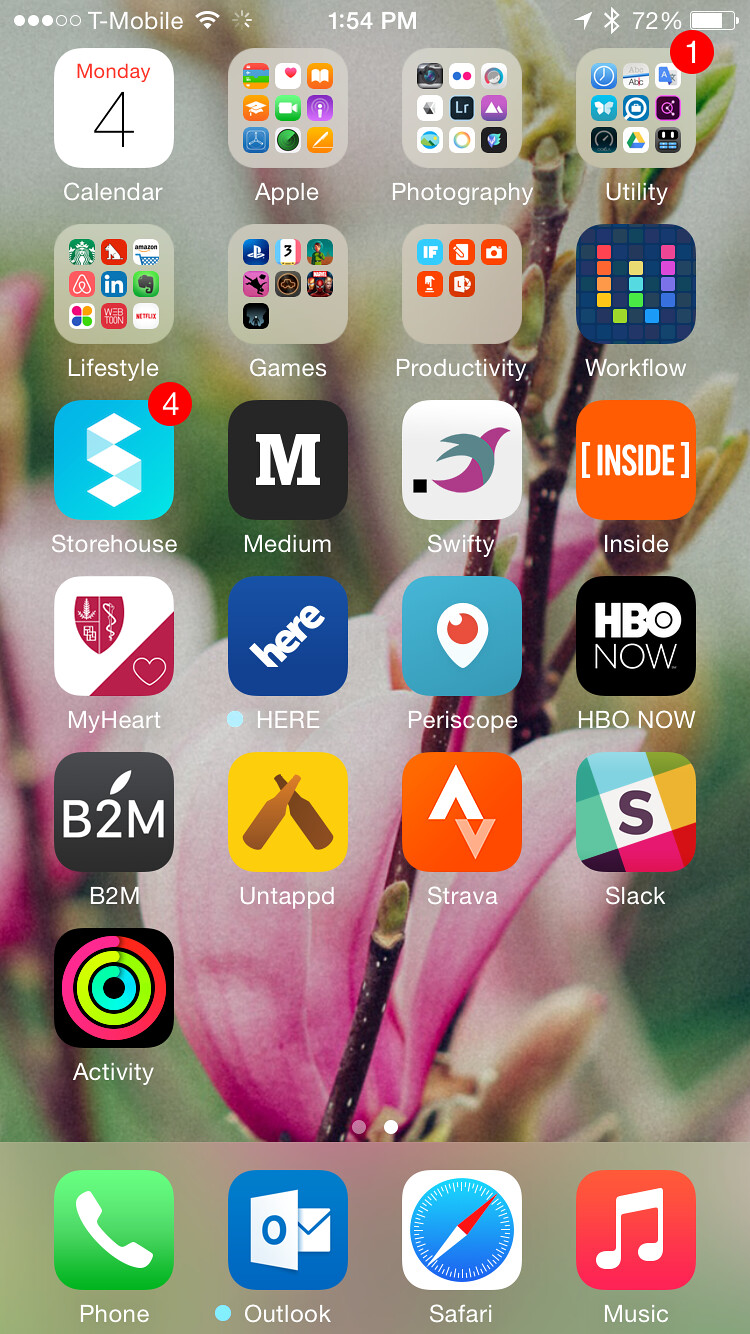This is a color photograph resembling a screenshot from a smartphone's home screen. It displays the main interface upon unlocking the device. The status bar at the top reveals that the service provider is T-Mobile, with full reception bars and the time set at 1:54 PM. The Bluetooth connection is active, and the battery level is at 72%, accompanied by a battery icon.

Beneath the status bar, the home screen is adorned with a variety of app icons. These include standard Apple apps, a range of photography apps, utilities, lifestyle applications, games, productivity tools, and workflow-related apps. Notably featured is an app named Storehouse, which currently has four notifications. Other highlighted apps include Medium, Swifty, Inside, My Heart, Here, Periscope, HBO Now, B2M, Untappd, Strava, Slack, and an activity tracker app. 

At the bottom of the home screen, there is a dock with essential apps such as the phone app, Outlook for email, the Safari web browser, and a music application.